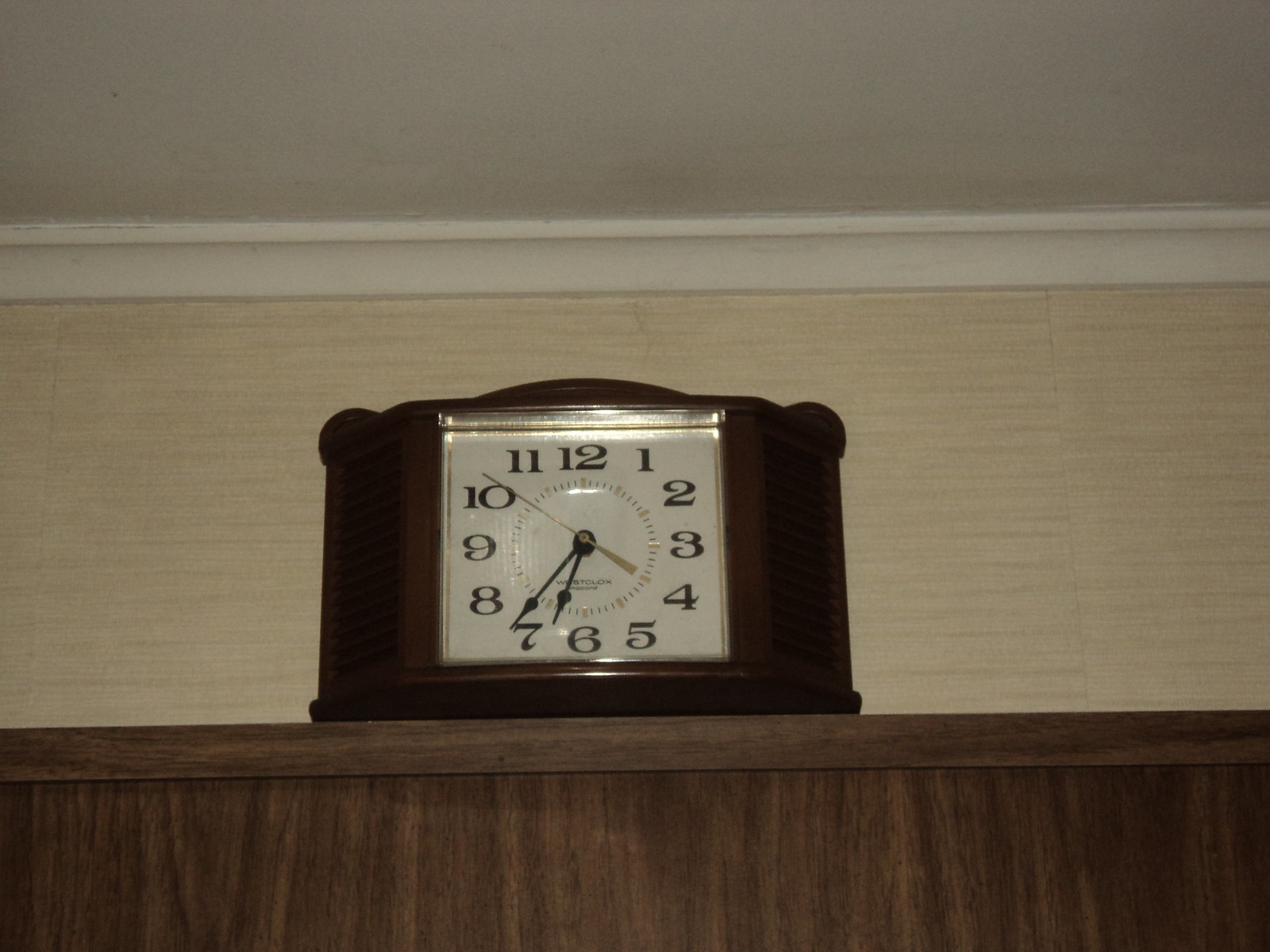The image depicts a wall adorned with a sophisticated white fabric wallpaper, resembling the pristine white edge at the top near the ceiling. Beneath this section, there's a contrasting dark brown area which appears to be made of wood, adding a rich warmth to the decor. This wooden section seamlessly transitions into a clock face, crafted from cloth and framed by a sleek black border. The clock features dash marks around its circumference and has twelve distinct increments, each precisely placed. The second hand of the clock is positioned between the 10 and 11 markers, while the hour hand is at the 8, and the minute hand lies between the 6 and 7 markers. Reflective light highlights the clock, adding a subtle glow to the white fabric portions, both on the left and at the top. Adding to the elegance, there's a trim of white wood at the top of the brown wooden section, enhancing the overall aesthetic with a touch of brightness.